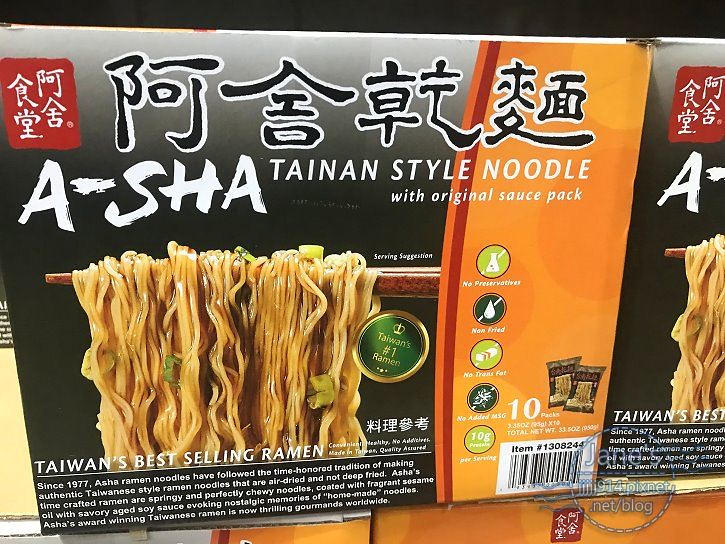The image depicts a box of ramen noodles, prominently displayed among other boxes in what appears to be a grocery store setting. The backdrop features a black and gray design with Chinese text outlined in white. Central to the imagery is the A-SHA Tainan-style noodle packaging, showcasing a vivid picture of wooden chopsticks lifting a generous portion of ramen noodles, complete with green onions, shallots, and a hint of brown broth. Dominating the packaging is a circular green logo with a gold border that proclaims, "Taiwan's number one ramen." 

The orange right side of the packaging includes several icons emphasizing the product's health benefits—no preservatives, non-fried, no trans fat, no added MSG, and 10 grams of protein per serving. White text on the bottom left announces, "Taiwan's best-selling ramen," and a descriptive paragraph underneath details the noodle's storied history, noting its popularity since 1977.